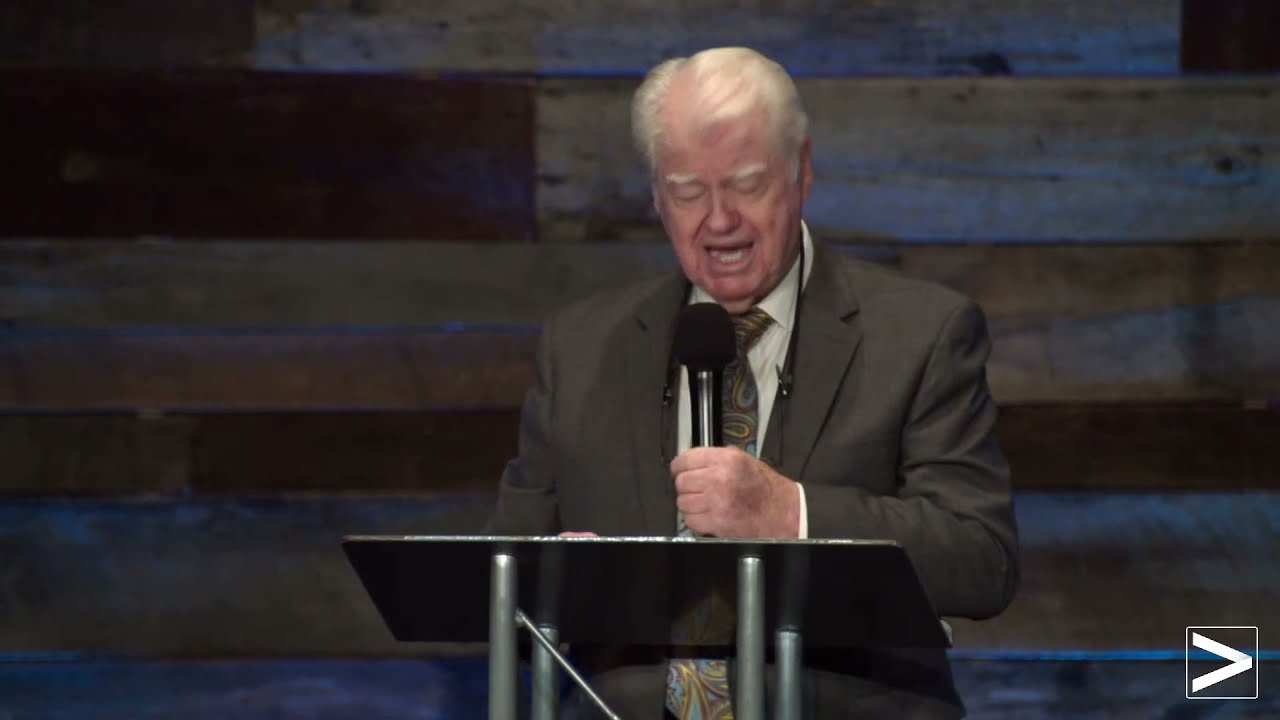The photograph captures an elderly white man, partially balding with white hair, delivering a speech from a podium in an indoor setting. He wears a dark brown suit, a white shirt, and a colorful patterned tie. He is holding a microphone in his left hand up to his mouth as he looks down at the material on the podium before him. Behind him, the background features a wooden wall composed of wide panels varying in tan shades, highlighted by some mood lighting. In the bottom right corner of the image, a white logo resembling a rotated V shape is visible, framed within a white-bordered square.